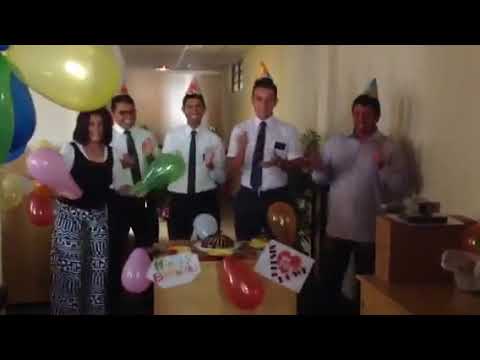This blurry, grainy image captures a cheerful birthday celebration, likely taking place at an office. Five people are shown, four of whom are men, with a woman standing on the left. The men in the middle wear white shirts and black ties, accessorized with pocket protectors, and the man on the far right dons a gray long-sleeve shirt. All the men, except perhaps the woman obscured by balloons, wear party hats. The woman is dressed in a black tank top layered over a white shirt and patterned black-and-white pants, holding a green and a pink balloon.

Balloons in various colors — including large yellow, blue, and green ones — fill the scene, with some visible in the top left corner. These balloons are round and elongated in shape. There appears to be a cake in the center, possibly on a table or box, surrounded by the group who are all sporting great big smiles. A sign, partially obscured, seems to say "Happy Birthday," adding to the festive atmosphere. The image is bordered in black at the top and bottom, framing the lively yet somewhat indistinct snapshot of the celebration.